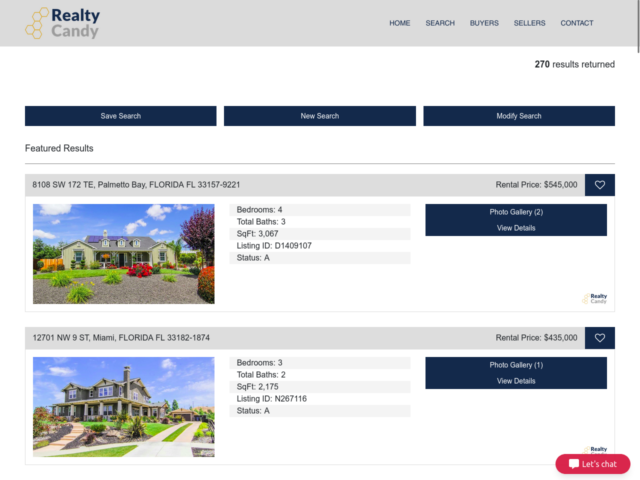The website interface of Realty Candy features a distinctive logo comprising five interconnected hexagons. The top banner, rendered in gray, displays "Realty" in dark black text and "Candy" in a slightly darker shade of gray, accompanied by muted gold hexagons. The navigation menu includes options for Home, Research, Buyers, Sellers, and Contact. The search yielded 270 results. Below the banner, three black tabs are labeled "Save Search," "New Search," and "Modify Search," followed by a section highlighting "Featured Results." The current search appears to focus on housing options in Miami, Florida, or Palmetto Bay. Two prominent listings are displayed: 

1. A 4-bedroom, 3-bathroom home with approximately 3,100 square feet, priced at $545,000. It is marked with a status "A" and includes a photo gallery as well as detailed viewing options.

2. A 3-bedroom, 2-bathroom home with around 2,200 square feet, listed for $435,000. Further details and photos are accessible for both properties.

This search indicates that someone is actively house hunting.